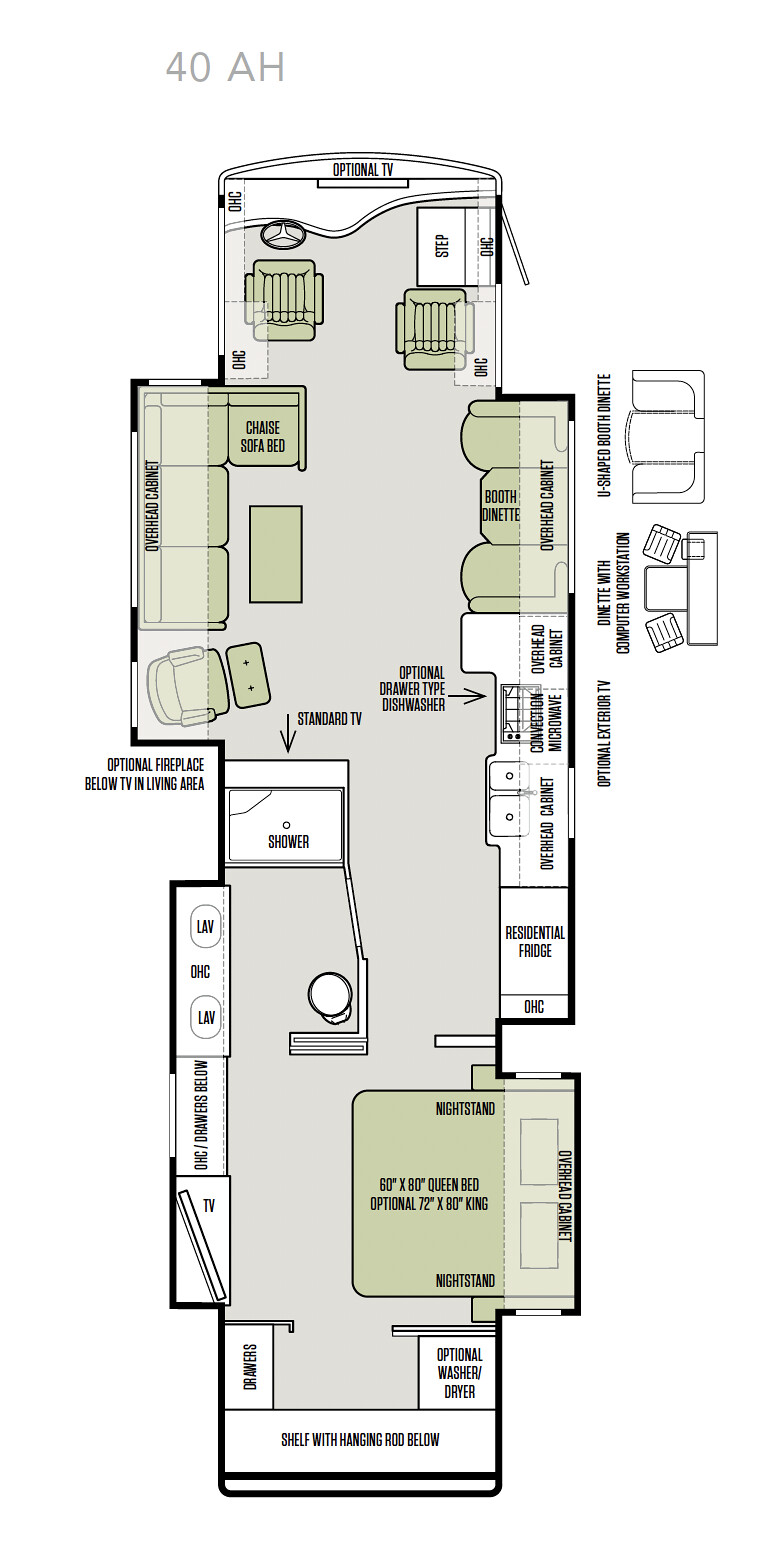This image depicts a detailed floor plan, likely for a boat, illustrating various sections and furnishings within a narrow, rectangular layout. At the top of the diagram is a sketch of a chair, square in shape and marked with lines, in front of what appears to be a steering wheel, hinting at the boat's helm. Adjacent to this helm station is another similar chair. Progressing further down the layout, a sequence of furniture is drawn: a couch accompanied by a rectangular table, an armchair paired with an ottoman, and opposite these, a clearly marked kitchen area featuring a sink. Continuing toward the end of the diagram, the layout includes a double bed, complete with two pillows. The meticulous representation of these sections and furnishings suggests a well-thought-out design intended for comfortable and functional onboard living.